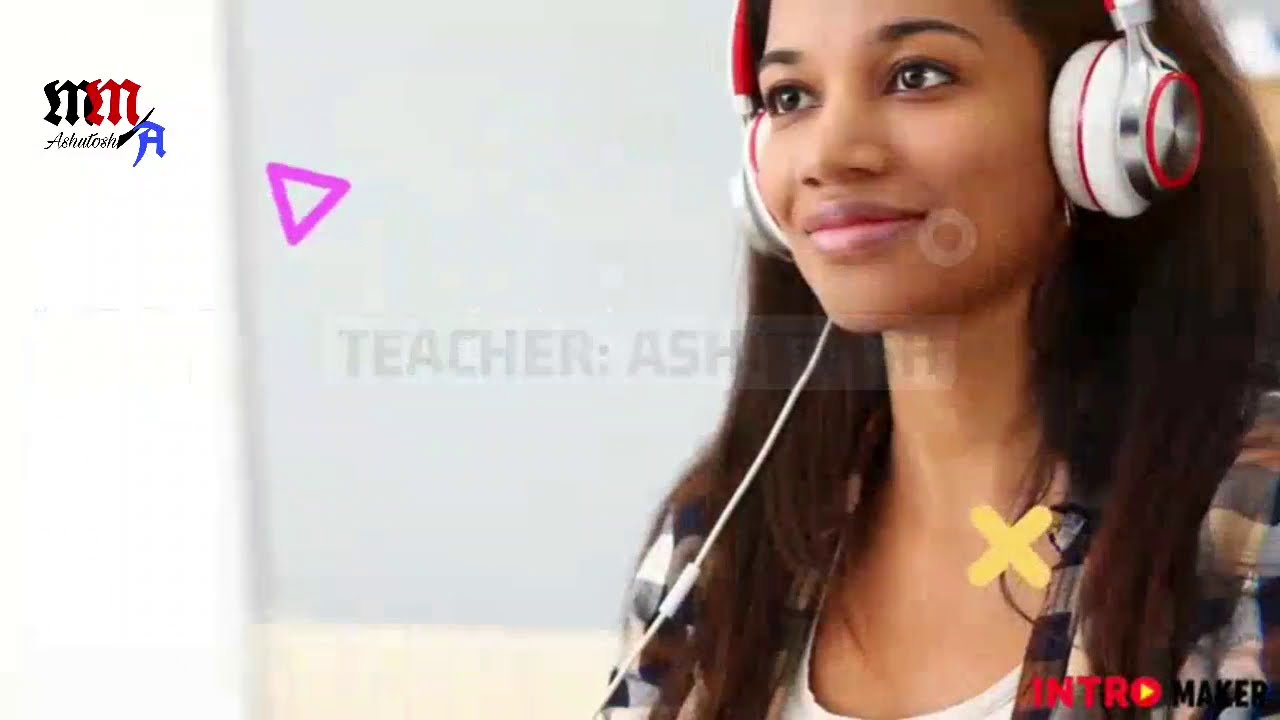The image features a brown-skinned young woman with brown eyes and slightly smiling closed lips, facing towards the left. She has brown hair that extends just below her shoulders and is wearing a black and tan flannel shirt over a white shirt. On her head, she sports large white headphones with red circles. Faintly visible at the corner of her mouth is a white mark resembling the letter "O."

At the base of her neck, a yellow "X" is prominent, with the word "INTRO" written in red underneath, where the "O" incorporates a yellow arrow pointing to the right. Following this, black text reads "MAKER." Across the center of the image, the word "TEACHER" followed by "ASH" is subtly visible but fades into the background.

On the left side of the image, there's a floating magenta triangle. Adjacent to this triangle is an emblem featuring the letters M (brown and red), a slash, and a blue letter A. Below the emblem, in cursive, it reads "ASHTENTECH." The photograph is horizontally oriented, with the woman placed on the right side of the frame.